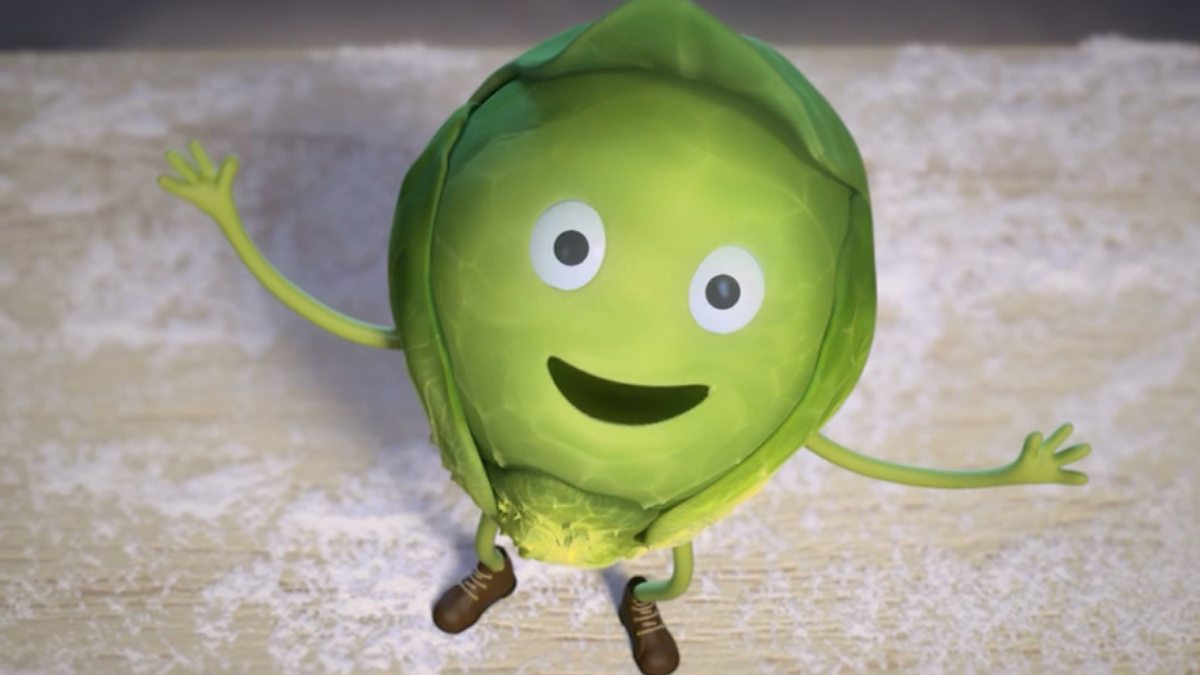In this detailed image, we see a lively, cartoon-style green character resembling a cabbage or Brussels sprout, viewed from slightly above. The character’s head is a vibrant green with vein-like leaf patterns, reminiscent of layered cabbage leaves. It has a friendly, happy facial expression with large, round white eyes and black pupils, accompanied by a wide, black smile. Green arms extend outward from its sides, as if offering a hug. Its thin, green vine-like legs lead down to brown leather shoes with white laces. The character stands firmly on a light-colored butcher's board, which displays a distressed, rustic appearance. Scattered across the board are small piles of salt, adding texture and context to the scene. In the background, the butcher's board transitions into a darker shade at the top of the image, enhancing the depth and contrast of the overall picture.